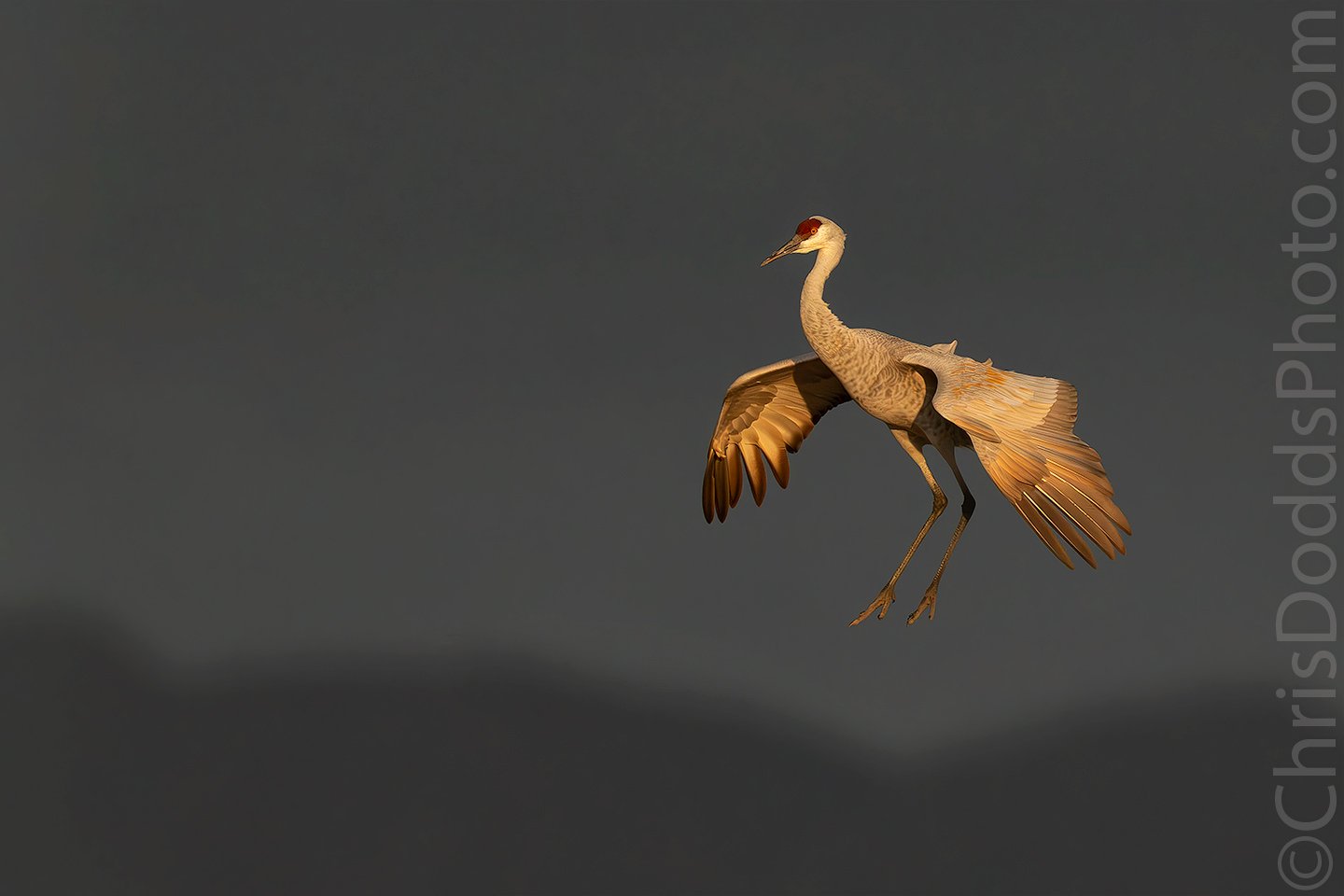In this striking image, we see a crane-like bird, possibly in mid-flight, meticulously set against a dark, shadowy background. The bird features distinctive red markings around the top of its head and eyes, creating a mask-like appearance. Its feathers are an array of colors, blending from black at the tips to various shades of brown, yellow, tan, and off-white. The bird's wings are outstretched, with the upper parts predominantly white and the lower parts transitioning to a darker hue. Its long legs dangle beneath it, showing the two visible toes on each foot. The background is an indistinct, blurred blend of black and gray, possibly suggesting a dark sky or water, with faint silhouettes of trees or mountains. Off to the side, the watermark "© chrisdoddsphoto.com" is visible in light gray font, vertically oriented to the right of the bird, ensuring credit to the photographer. The overall effect is dreamlike, as if the bird has been expertly captured in motion, yet there’s an air of careful composition that suggests it might also have been photoshopped.